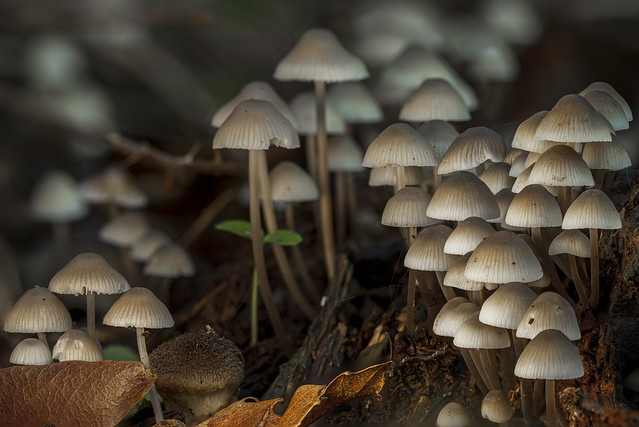This photograph captures a close-up of a woodland scene, focused on a cluster of small, white mushrooms with slightly darker, thin stalks emerging from dark soil. The mushrooms, which have pleated dome-shaped caps, display delicate, thin tendrils underneath, resembling tiny white umbrellas. The scene is characterized by a mix of colors and textures, with a prominent brown leaf in the foreground, its individual veins and striations visible, suggesting it is old and crunchy. Among the mushrooms, a few green weeds sprout up, adding a touch of freshness to the otherwise dark and earthy setting. The image's background is a blurred mosaic of greens and whites, accentuating the main subjects and giving the photograph a dreamy, natural ambiance.